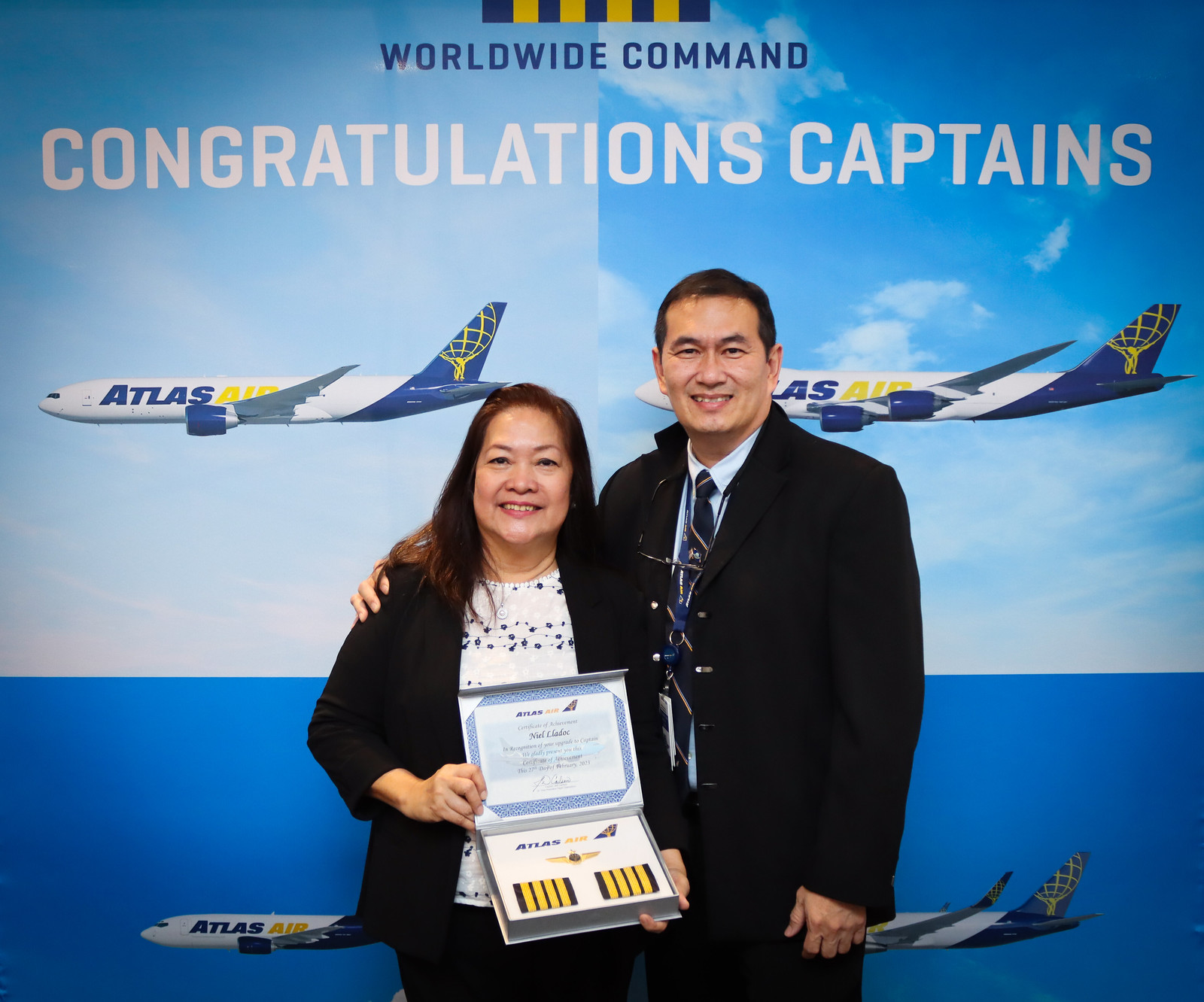In the photograph, two middle-aged individuals of Asian descent stand proudly in front of a banner. The banner prominently displays the words "Worldwide Command" in dark blue at the top center and "Congratulations Captains" in larger white font just below. The backdrop showcases four scenes of the same Atlas Air airplane—a mostly white aircraft with white wings, a blue tail, and tail fins adorned with a yellow depiction of the Greek god Atlas holding up the earth. Each scene depicts a different sky: one with thin white clouds, another with wispy clouds, and the bottom two with clear blue skies.

The woman, standing to the left, has long brown hair and is dressed in a white blouse with a floral black design, a black jacket, and black pants. She holds a certificate in a box, bearing the Atlas Air logo and epaulets with four stripes each. The man to her right, a head taller, has his arm affectionately around her. He is dressed in a light blue shirt with a tie, a dark jacket, and black pants. Both are smiling, and the celebratory and formal atmosphere suggests they have been recognized for an achievement, possibly in aviation, as indicated by the details on their attire and the congratulatory banner behind them.